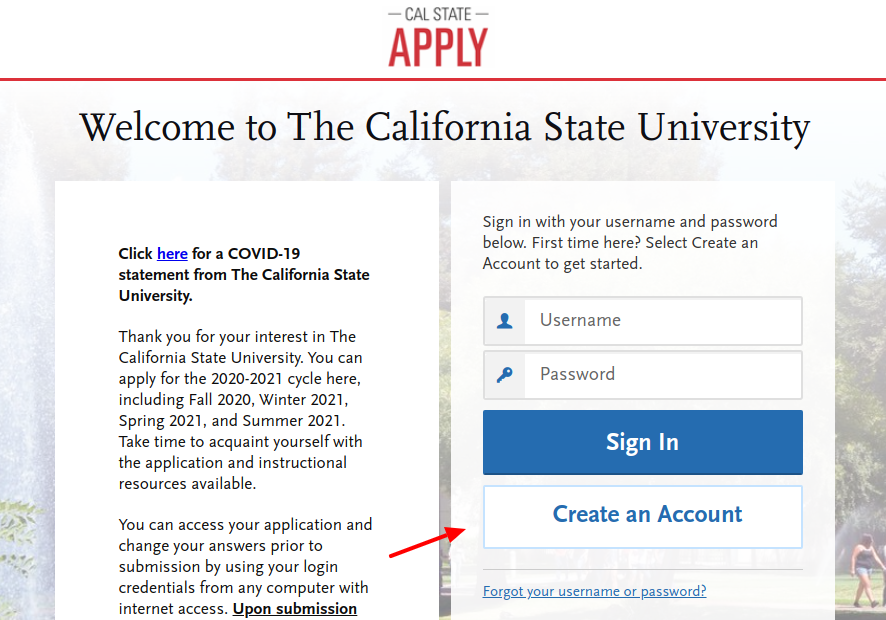The top of the registration page for a California State University account prominently features the header "Cal State." Directly beneath this is the word "Apply" in large, red letters. Underneath, it welcomes users with the phrase "Welcome to the California State University."

On the left column, a message reads, "Click here for a COVID-19 statement from the California State University." This is followed by text thanking applicants for their interest in the university and informing them that they can apply for the 2020-2021 academic cycle, which includes Fall 2020, Winter 2021, Spring 2021, and Summer 2021. The message encourages applicants to familiarize themselves with the application process and available resources, and mentions that they can access and modify their application answers prior to submission using their login credentials from any internet-connected computer. The text further detailing what happens upon submission is cut off.

A red arrow on the left side of the page points to the right-hand column. This column contains instructions for signing in with an existing username and password, and guides first-time visitors to select "Create an account" to begin the registration process. 

Below these instructions, there is a rectangular input box featuring an icon of a person's head with the placeholder text "Username" inside it. The subsequent input box displays an image of a key followed by the word "Password." There is also a blue rectangular button with the text "Sign In" centered in white, and another rectangular button with a white background that reads "Create an Account" in blue text. 

At the bottom of the page, there is a link for users who have forgotten their username or password.